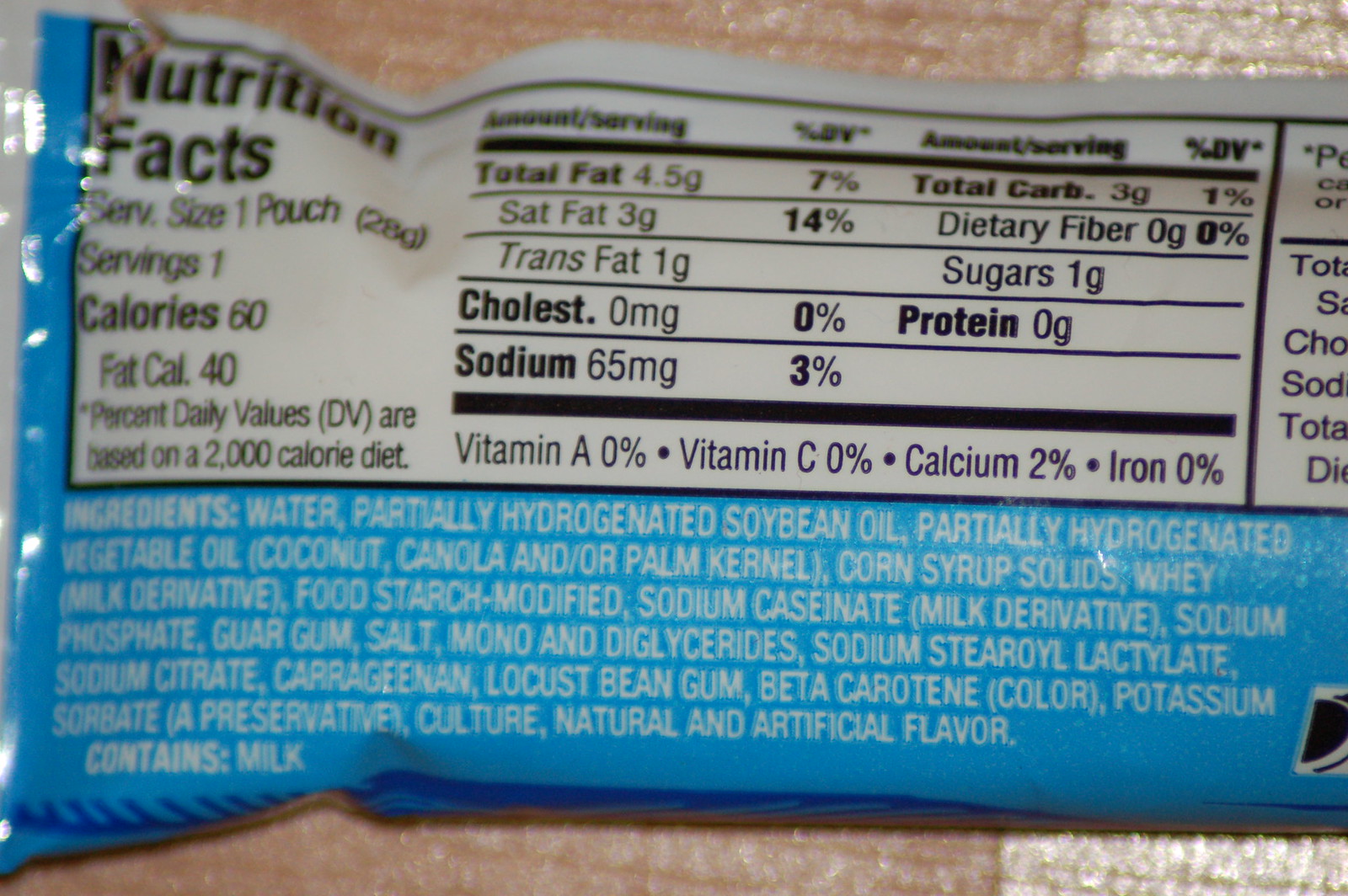The photograph captures the nutrition facts on the back of a blue food package. The nutrition information is presented within a white inset, making it clearly visible. The package lists the serving size as one pouch, weighing 28 grams, and states that there is only one serving per package. Each serving contains 60 calories, with 40 of those calories coming from fat. The total fat content is 4.5 grams. Additionally, the package lists total carbohydrates at 3 grams, and notes that it contains 0 grams of protein. Key ingredients include water, partially hydrogenated soybean oil, partially hydrogenated vegetable oil, corn syrup solids, and whey. The detailed nutrition facts and ingredients suggest that the product is a processed food item.